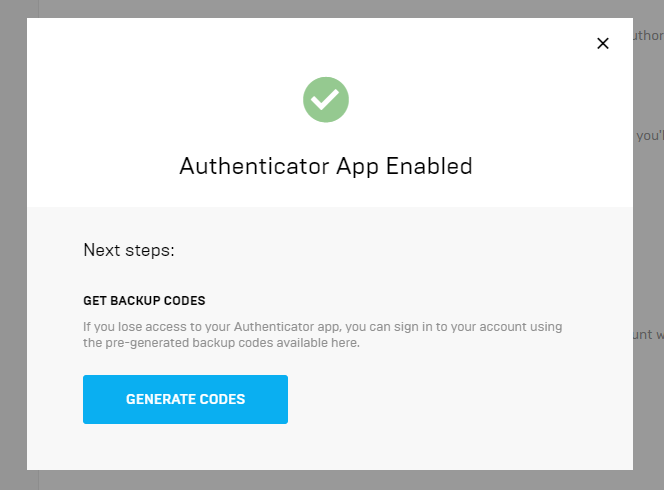The image depicts a user interface with a grey background, overlaid by a large white dialogue box occupying most of the screen. In the upper right corner of this dialogue box, there's a small 'X' symbol for closing the window. Centrally located within the dialogue box is a green checkmark, signifying a successful action. Beneath this checkmark, black text on a white background reads: "Authenticator app enabled."

At the bottom of the dialogue box, there is a light grey panel providing additional instructions. This panel advises the user on the importance of obtaining backup codes, stating: "If you lose access to your Authenticator app, you can sign in to your account using the pre-generated backup codes available here." Following this message, there is a blue, rectangular button with white, uppercase text that reads "GENERATE CODES."

The primary purpose of this dialogue box is to confirm that the Authenticator app has been successfully enabled by the user. Additionally, it serves as a precautionary reminder, urging the user to generate and store backup codes. These codes will allow the user to regain access to their account in the event they lose access to their Authenticator app.